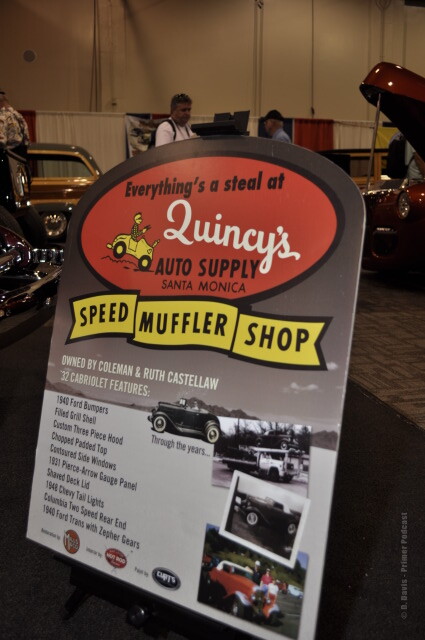The image captures an indoor scene, likely at a car show held in a convention center or warehouse, evidenced by the wood flooring and red and white curtains in the background. Antique and classic cars are partially visible on either side, including a distinctive red car with its hood up and the back end of an old station wagon featuring wood paneling. The scene features at least three people, including an old man wearing a hat and a man in a white t-shirt with a backpack. The central focus of the image is a prominent cardboard sign with a gray top half and white bottom half. The sign reads in black letters on a red background: "Everything's a steal at Quincy's Auto Supply Santa Monica." Below, a yellow banner displays the words "Speed Muffler Shop." The sign features a red oval with the same text and includes a small illustration of a man in a car. Additional text on the sign provides details about various vintage vehicles, including: "Owned by Coleman and Ruth Castellaw. 32 Cabriolet features 1940 Ford bumpers, fixed grille shell, custom three-piece hood, chopped padded top, corseted side windows," accompanied by photographs of these classic cars.